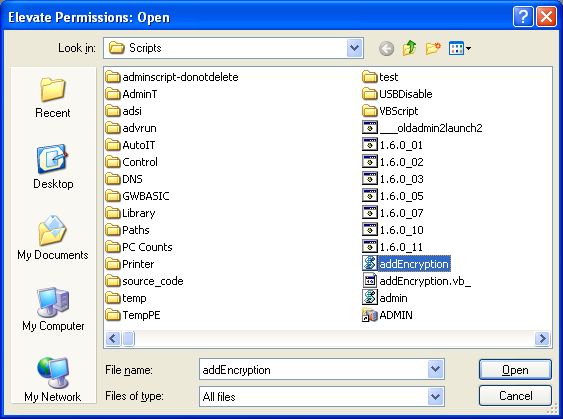This is a detailed screenshot from a Windows XP computer displaying a typical file navigation window. The interface features a characteristic blue bar at the top with the text "Elevate Permissions: Open" along with a question mark button and a red X button for closing on the right. Below this is a gray-bordered area labeled "Look in," accompanied by a folder icon and a drop-down arrow next to the word "Scripts."

On the left side of the window, there is a vertical navigation pane listing several directory options with corresponding icons: "Recent," "Desktop," "My Documents," "My Computer," and "My Network." These directories aid in quick navigation through commonly accessed folders.

The main central area has a white background filled with icons of folders displayed in a grid-like arrangement, identified by their names. One of these folders, named "Add Encryption," is highlighted, suggesting that it has been selected for opening.

At the bottom of the window, there is a "File name:" field indicating "Add Encryption" and a drop-down menu labeled "Files of type," currently set to "All files." The bottom right corner houses two buttons— "Open" and "Cancel"— for executing or aborting the command, respectively. The overall screenshot captures the user interface for managing files in a clear and organized manner on a Windows XP system.